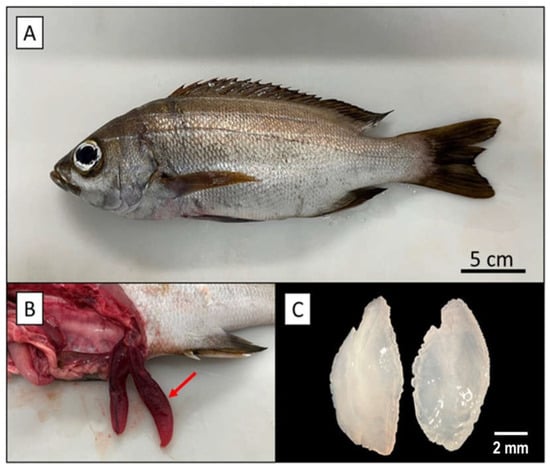This composite image, possibly from a scientific journal, consists of three distinct panels showcasing a fish and its internal structures. 

The top, largest panel labeled "A," features a side view of a deceased fish. It rests on a light gray background with a darker gray shadow, enhancing its three-dimensional appearance. The fish, grey and silver with black-tipped fins and tail, lies on its right side, facing left. A measurement scale at the bottom of the panel indicates the fish is 5 centimeters long. 

The bottom left panel, labeled "B," half the height of the top panel, presents a dissection of the same fish. This image reveals the fish's gutted belly, exposing internal organs. Blood and other internal matter are visible, emphasized by a red arrow pointing to two red, elongated shapes hanging from the fish's abdomen. 

The smaller bottom right panel, labeled "C," is set against a black background. It shows two white, translucent, oval structures, which appear gelatinous and measure 2 millimeters each, as indicated by the scale beneath them. This panel may depict close-up views of internal fish structures or scales.